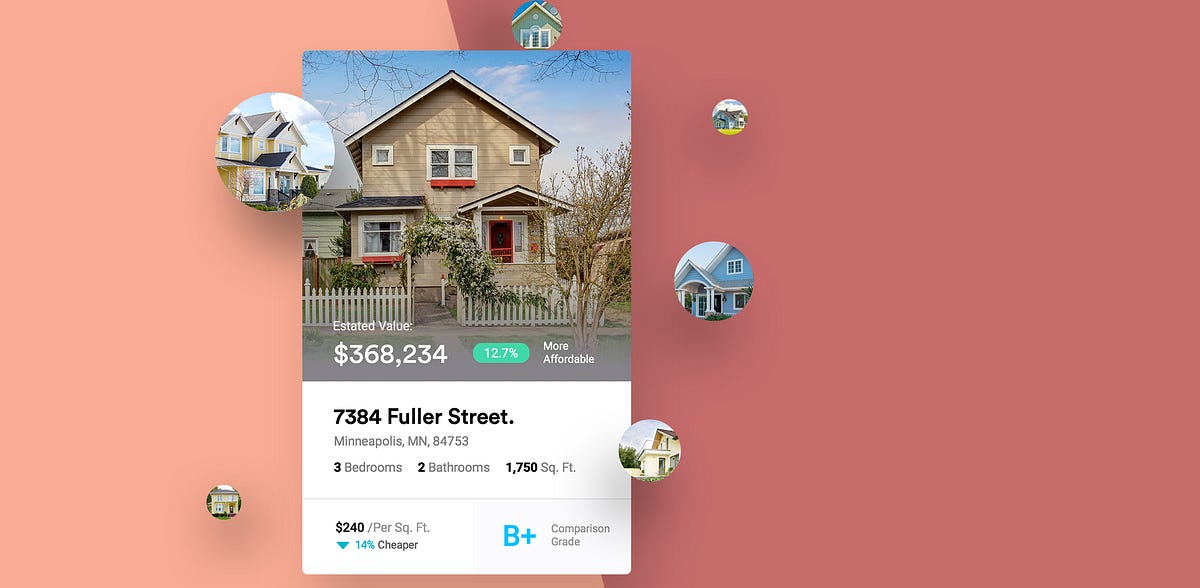The image features a large rectangular area spanning from the right edge to the middle of the composition, transitioning from a dark peach shade on the right to a lighter peach shade on the left. At the center, where these two colors converge, there is an inset picture of a two-story house. The house is light brown with beige undertones, featuring a V-shaped roof. 

On the top left of the house, there is a small window, and a larger, double window sits in the middle, adorned with a flower box that has orange flowers. Additionally, there is a small window on the right. Beneath the middle window, an awning extends above a large window situated on the left side of the house, which also has orange accents under it. All the windows are trimmed in off-white. The front door, painted orange and framed in white, opens out to a small porch with a railing and is bordered by a white picket fence. Additional structures of the house, potentially the garage, are visible on the left side.

Above the house image, the text "Estimated Value" is displayed, followed by "$368,234." Positioned on a green banner nearby, the text "12.7% more affordable" is written in white. Below the house image, detailed information about the property is provided: "7384 Fuller Street, Minneapolis, Minnesota, 84753." It highlights that the house has three bedrooms and two bathrooms, encompassing 1,750 square feet, with a cost of $240 per square foot. An accompanying green arrow with "14% cheaper" in green text indicates its relative affordability. 

Additional details include a "B+" in blue, labeled as "Comparison Grade" in gray text, along with small circular images of different houses. These house images are arranged in a sequence with one at the top, another on the left, and three more on the right, showcasing various two-story houses, possibly condos.